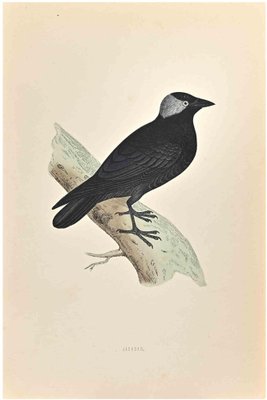This is an illustration reminiscent of an old Audubon-style bird depiction, set against a worn, beige paper background. The focal point is a black bird, likely a crow, perched on a diagonally positioned branch that cuts from slightly above the left-center to slightly above the bottom-right of the paper. The branch has a lighter beige color, accentuated by blue and darker highlights, and features a small, pointy twig extending from near its bottom-left. The bird, standing near the branch's lower part, is depicted in meticulous detail: it sports a body covered in black feathers, black taloned feet, and a sharp black beak. Notably, a gray triangular marking extends from the bird's eye—a gray eye with a black pupil—towards the back of its head. The bird's profile view, showcasing the separate feathers on its wings and tail, adds to the realism. Near the bottom of the picture, there is a small line of gray text that is illegible.